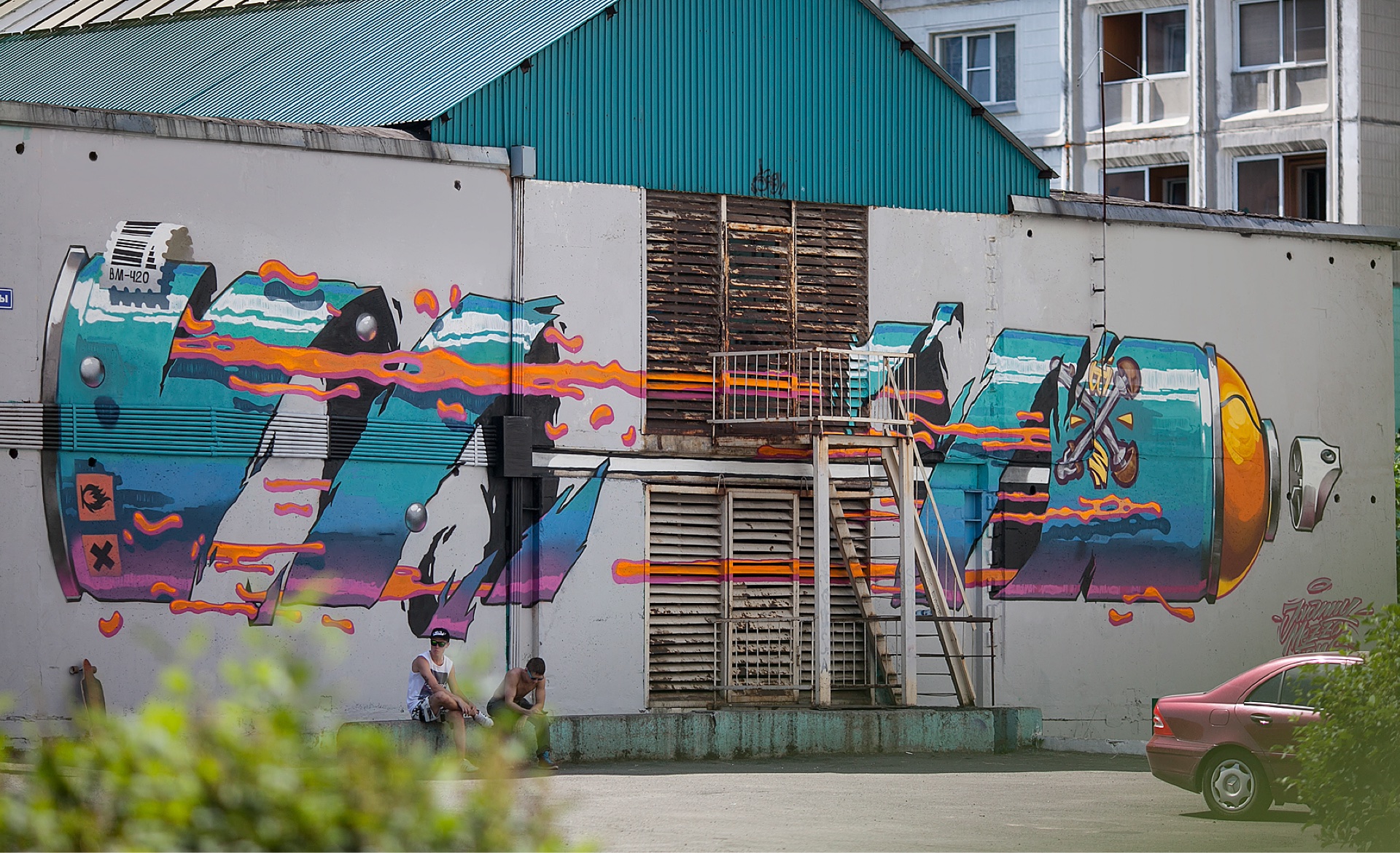The image captures a vibrant and colorful mural painted on the side of an industrial-style apartment building. The mural, predominantly in shades of blue, teal, and orange, creates a dynamic contrast and extends from the left to the right side of the frame. Central to the composition is a long, cylindrical object resembling an aerosol can that appears cut into a spiral shape. The can is intricately detailed, with a turquoise hue matching parts of the building’s metal roof and rooftop, and features elements like a white aerosol sprayer and an orangish top. 

Orange and pink wavy stripes extend across its length, giving the impression of fluid escaping from it. The mural cleverly integrates the architectural features of the building, such as windows and vents, which become part of the artwork, and a set of wooden louvers within the cylindrical object. The balcony with a railing overlaps part of the mural, adding depth to the scene. In the foreground, a red car and green shrubs are partially visible, adding context to the photograph’s setting. The vibrant colors and imaginative depiction invite viewers to engage with the narrative suggested by the interacting figures within the mural.